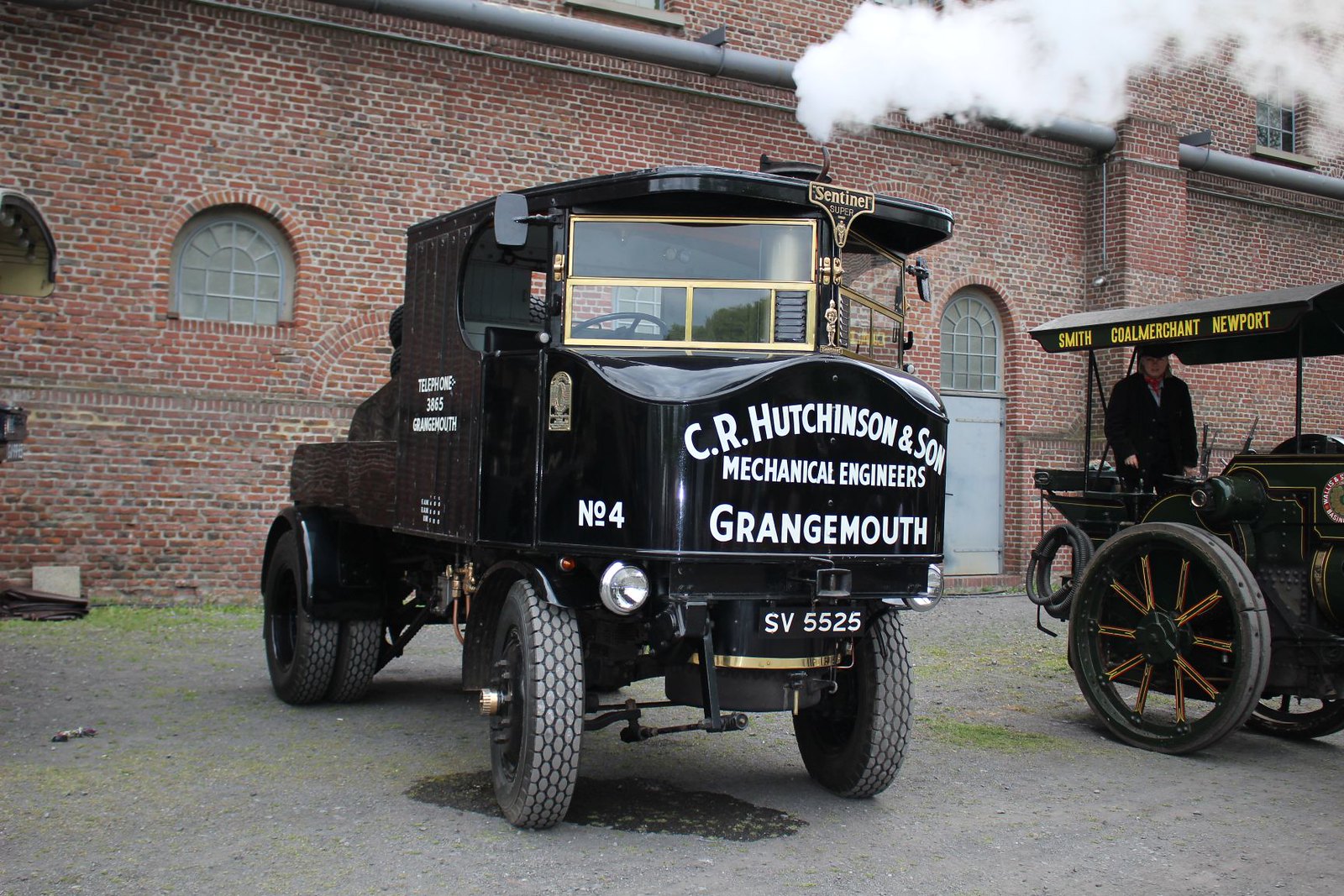This outdoor photograph captures two vintage black vehicles parked on a cement pad in front of a red brick building with several half-circle windows. The central focus is a large, antique delivery truck with gold-edged square windshields and tall, spoke wheels. Painted on the front of the truck, which seemingly belongs to "C.R. Hutchinson and Son, Mechanical Engineers" from Grangemouth, is the number "4" along with the license plate "SV5525." The vehicle features a flatbed section, hinting at its delivery use, and emits a wisp of smoke from a stack on top, trailing off to the upper right of the image.

To the right of this main truck is another black, vintage vehicle, partially cropped out of the frame. It further adds to the scene of historical nostalgia. This second vehicle bears the name "Smith Coal Merchant Newport" and is fitted with a canopy top and substantial spoked wheels. Nearby, a man stands at the back of this vehicle. The entire setting suggests a bygone era, possibly the 1920s or 30s, captured with detailed authenticity against the reddish-bricked, classic architectural backdrop.